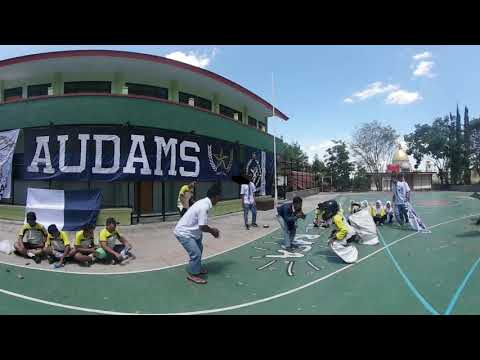Captured on a sunny day, this vibrant outdoor scene showcases a large, tall building on the left side with a blue banner bearing white text reading "ADAMS," and possibly misspelled as "AUD AMS." In front of this building, a track field or green concrete playground with white and blue lines stretches out. Seven to eight individuals, possibly school students from South Asia, are seated and engaged in creative activities, likely drawing with chalk on the ground. These individuals are mostly boys donning yellow, white, and black uniforms, suggesting a school setting. Sitting crisscross applesauce, some of them interact with a man in a white shirt and blue jeans who is bending down to engage with them. The background features a series of trees and a large, dome-shaped building partially hidden behind the trees, lending a picturesque quality to the landscape. Watching the activities unfold, a few people stand near the building, while under the blue sky dotted with clouds, the setting pulses with an atmosphere of education and youthful creativity.